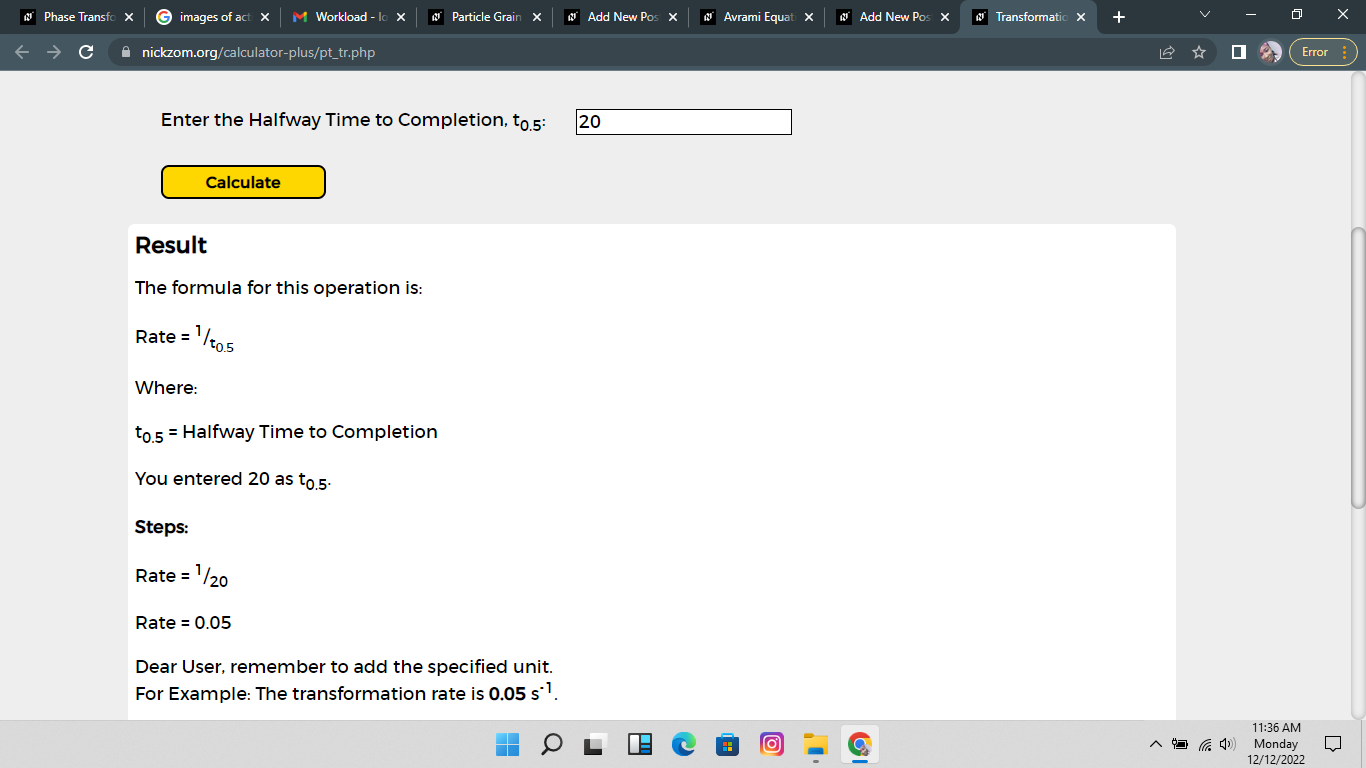**Image Description: Web Page Showing Calculation of Transformation Rate**

The image depicts a snapshot of a webpage with multiple open tabs, with emphasis on the currently selected tab labeled "Transformation." The main content area displays a form where users input data to calculate the transformation rate.

- **Main Content**: The form is asking the user to "Enter the halfway time to completion," represented by the notation T^0.5, which is a box where the user has entered the number "20". Just above this input box, a yellow button labeled "Calculate" is prominently placed.

- **Result Section**: Below the input area, instructions and formulae are listed. It states, "The formula for this operation is rate = 1 / (T^0.5)," wherein T^0.5 is specified as the halfway time to completion. The user-entered value ("20") is acknowledged in the context of the formula.

- **Calculation Explanation**: The next section provides step-by-step guidance:
  - The rate calculation example suggests using the value "1 / 20" to determine the transformation rate.
  - Clarification for the user: "Dear user, remember to add the specified unit. For example, the transformation rate is 0.05 s^(-1)."

- **Additional Interface Elements**: At the bottom of the page, icons for social media apps like Instagram are visible, indicating options for social sharing or further interaction. 

- **Navigation**: The webpage also has several other tabs, denoting additional sections of the website that could be clicked on, offering further functionalities or information.

The overall layout emphasizes user input and clear, prompt feedback for calculating scientific data, incorporating user-friendly instructions and interactive elements like social media icons.